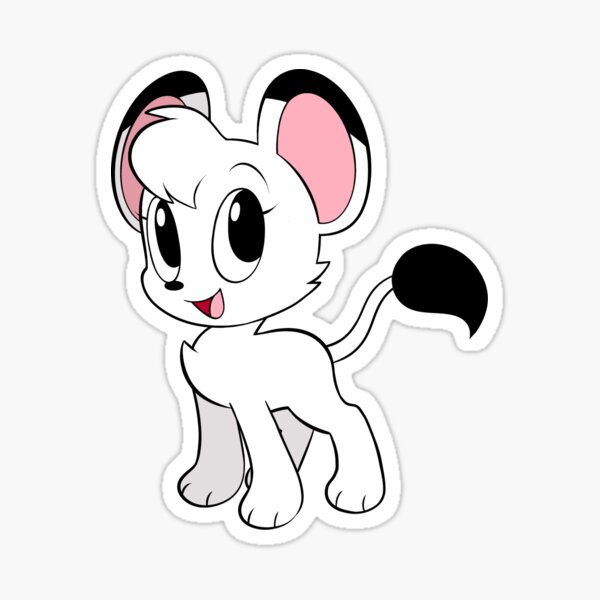This vibrant sticker features a charming cartoon dog set against a fully white background. The dog, primarily white in color, exudes a playful and cheerful demeanor, evident from its open mouth displaying a pink tongue and the red and pink accents suggestive of its mouth's interior. The dog's most notable features include its large, expressive black eyes with prominent eyelashes, suggesting a female character. The dog's ears are notably large, with black tops, gray and white bases, and pink inner centers. A distinct white fringe gives the appearance of hair or bangs, adding to its endearing charm. The dog has a small black button nose. Furthermore, its tail, mostly white, has a fluffy black end. While its body and two legs are white, the other two legs are gray. Overall, this detailed and animated depiction captures a happy and playful essence, manifesting in a cute and appealing anime-style character.